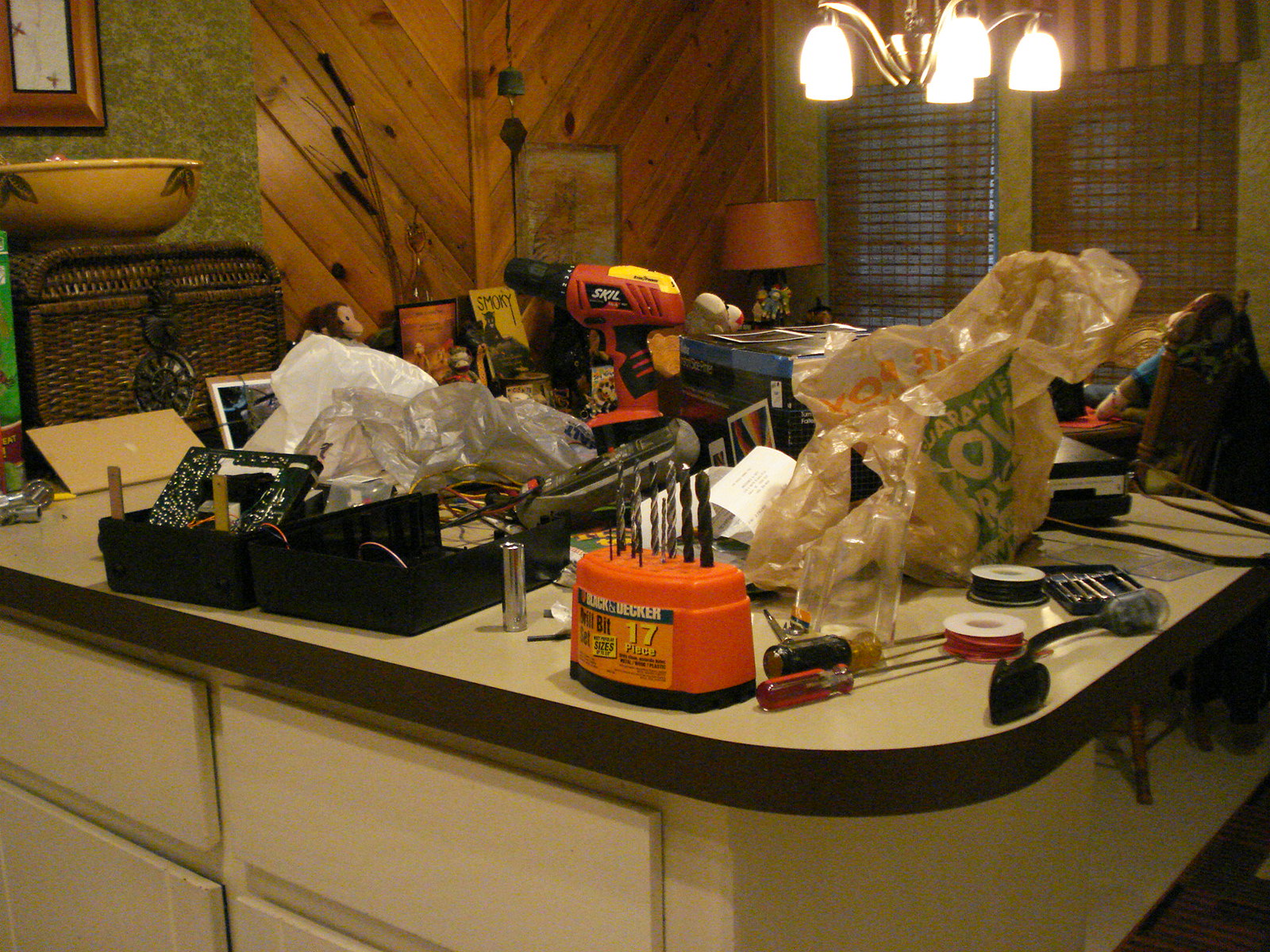This image captures a bustling kitchen scene where a white countertop with a black band along the edge serves as the focal point. The countertop is currently strewn with an array of tools including screwdrivers, drill bits, and electrical tape, indicative of an ongoing home project. A grocery bag from Home Depot contains additional supplies, adding to the cluttered workspace.

The cabinets and drawers beneath the countertop are a clean, crisp white, aligning with the overall kitchen aesthetic. In the background, the room transitions into a dining area identifiable by a table positioned beneath a chandelier. The walls here feature a distinctive wood paneling arranged in a sophisticated herringbone pattern, adding an element of elegance to the space.

Noteworthy details include a striking green marble pattern on the wall behind the counter, creating a visually appealing backdrop to the scene. Additionally, an antique ceramic bowl placed on the counter stands out amidst the tools, adding a touch of charm and history to the otherwise contemporary kitchen environment.